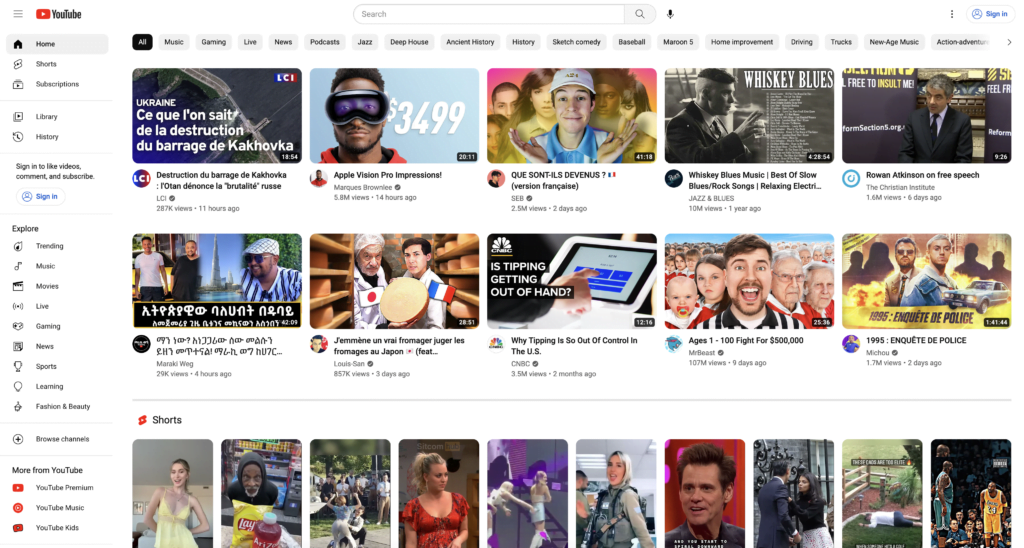The YouTube homepage is displayed, featuring the iconic red YouTube logo at the top. The navigation menu on the left includes highlighted 'Home', 'Shorts', and 'Subscription' buttons, with the 'Home' button currently selected and shaded in gray. Below that, there are options for 'Library,' 'History,' and a prominent blue 'Sign In' button. The menu also offers an 'Explore' section where users can browse trending content across various categories such as music, movies, live streams, gaming, news, sports, learning, fashion, beauty, and channels. Additional sections include 'YouTube Premium,' 'YouTube Music,' and 'YouTube Kids' under the 'More from YouTube' category.

At the top center of the page is a search bar that allows users to type queries or use a microphone for voice search. On the far right, another 'Sign In' button is located. Below the main navigation bar, categories like 'All,' 'Music,' and 'Gaming' are available, with 'All' being currently selected and highlighted in black.

The main content area showcases rows of video thumbnails, each marked with the video's duration in the bottom right corner. The thumbnails provide a preview image, while underneath, there's a brief description, the uploader's name, the view count, and the video age. Featured videos include topics such as the war, possibly in Spanish or Ukrainian, as well as product impressions like the Apple Vision Pro.

At the very bottom, a series of 'Shorts'—brief, quick-consumption videos—are displayed with their own thumbnails. Each of these also features a preview image to entice viewers.